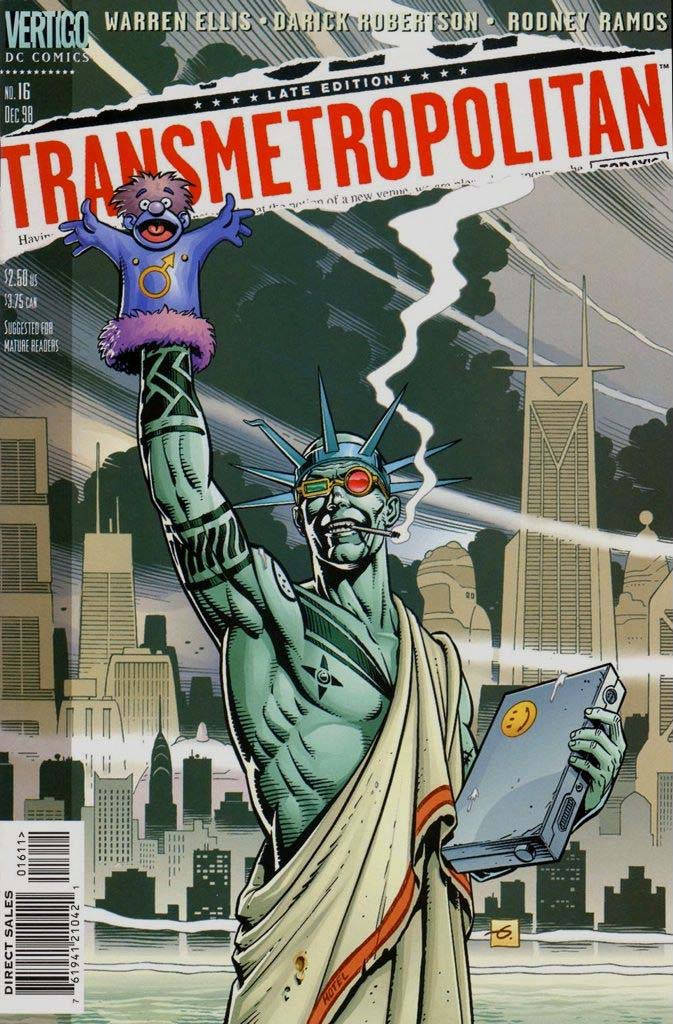This image is a vividly styled comic book cover, resembling an A4 format or magazine cover, titled "Transmetropolitan, Late Edition" in bright red letters at the top. The central figure is a satirical depiction of the Statue of Liberty, portrayed as a man adorned with tattoos on his arms and chest. He is smoking a cigarette, with the smoke spiraling upward and spreading across a detailed cityscape backdrop, which includes tall skyscrapers of New York. The man wears eccentric sunglasses, with one lens round and red, and the other rectangular and green. He is dressed in a toga and holding up a purple puppet in one hand, while carrying a suitcase in the other. Additional details on the cover include the words "Vertigo, DC Comics, Warren Ellis, Derrick Robertson, and Rodney Ramos," along with a barcode for direct sales scanning on the left side. In the background, beyond the city structures, blue skies and clouds are visible, adding depth to the image.